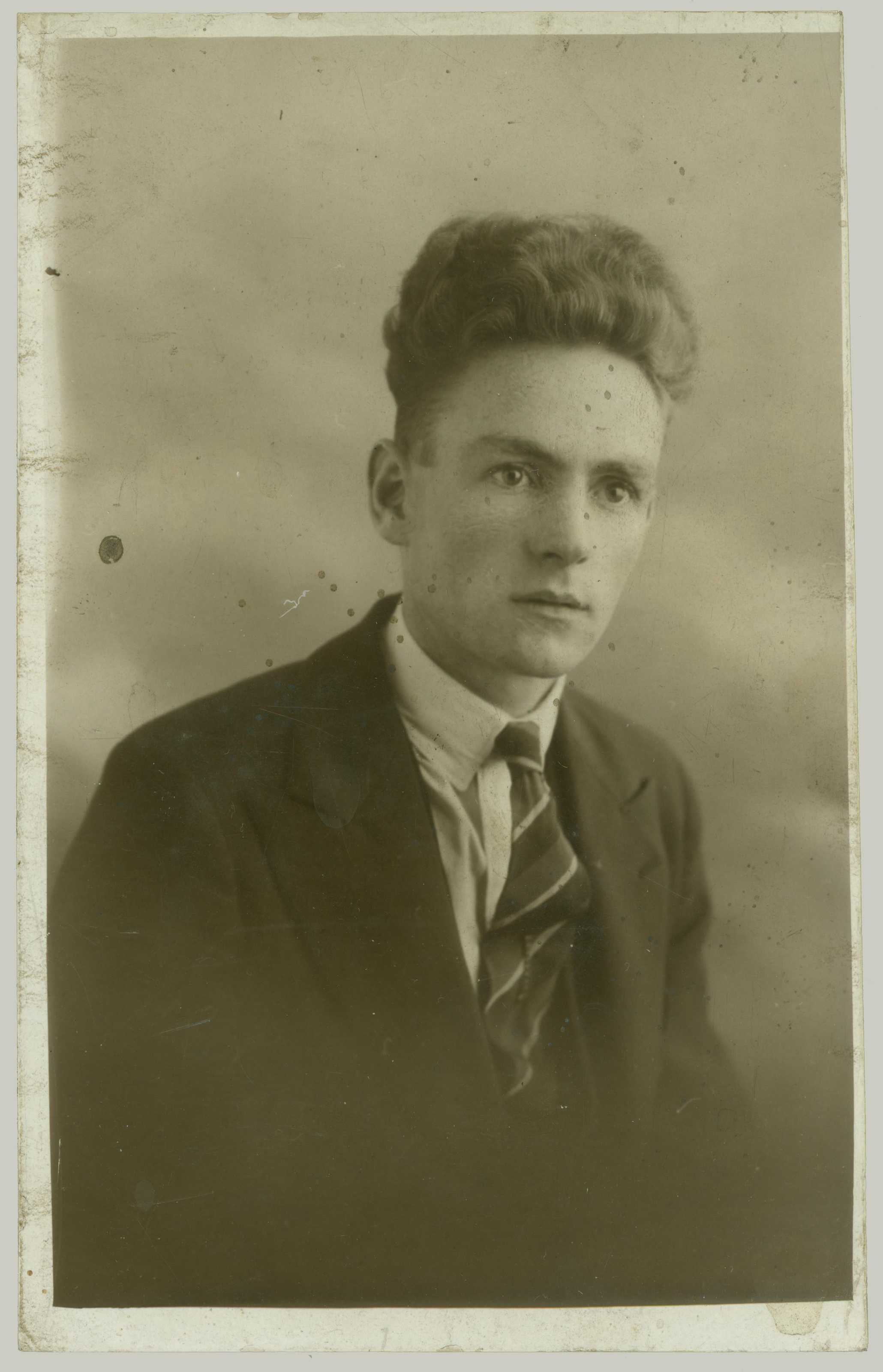This is a detailed black-and-white portrait photograph of a younger man, likely in his late 20s or early 30s, dressed in a charcoal suit with a striped tie and a button-up shirt. The man is seated and captured from the midsection up to the top of his head. Notably, his hair is styled interestingly: it is shaved on the sides but poofs up on top, giving it notable height, somewhat reminiscent of clouds, which is fitting given the cloudy background of the image. The photograph has a noticeable age to it, evidenced by its faded quality and various markings. The man is looking past the camera to the right, his shoulders slightly slanted, lending a contemplative mood to the portrait. Despite the ambiguity about whether it was taken indoors or outdoors, the lack of natural light and the formal composition suggest it was likely taken in a studio setting, focusing entirely on the individual without any accompanying text. The photograph is oriented vertically, being taller than it is wide, emphasizing the subject's poised posture and distinctive hair.